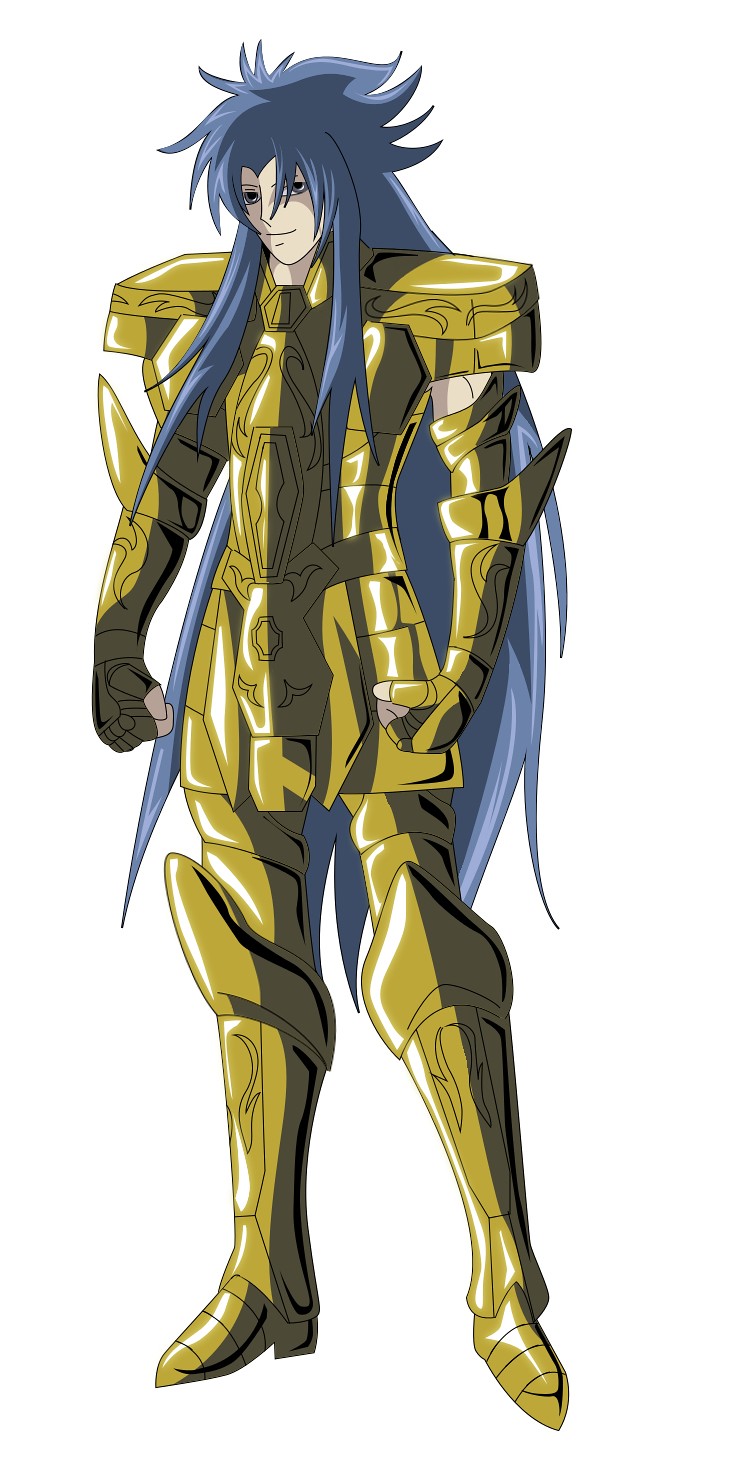The image depicts an anime character with very long, bluish-gray hair that extends down to the top of their calves, approximately three feet in length. The character is adorned in intricate golden armor that features a futuristic design. This armor is detailed with large, angular shoulder pads, spikes on the elbow area, and swirly engravings around the forearm shields. A symmetrical pattern runs from the center chest plate down to a hanging groin cover. The armor, which also includes boots extending past the knees, appears slightly damaged in places, adding to its worn, battle-ready appearance. The depicted character has pale skin and blue eyes, and the hair, while long at the back, is shorter and spiky on top, enhancing the overall anime aesthetic. The background is plain white, drawing complete focus to the character's elaborate and striking design.